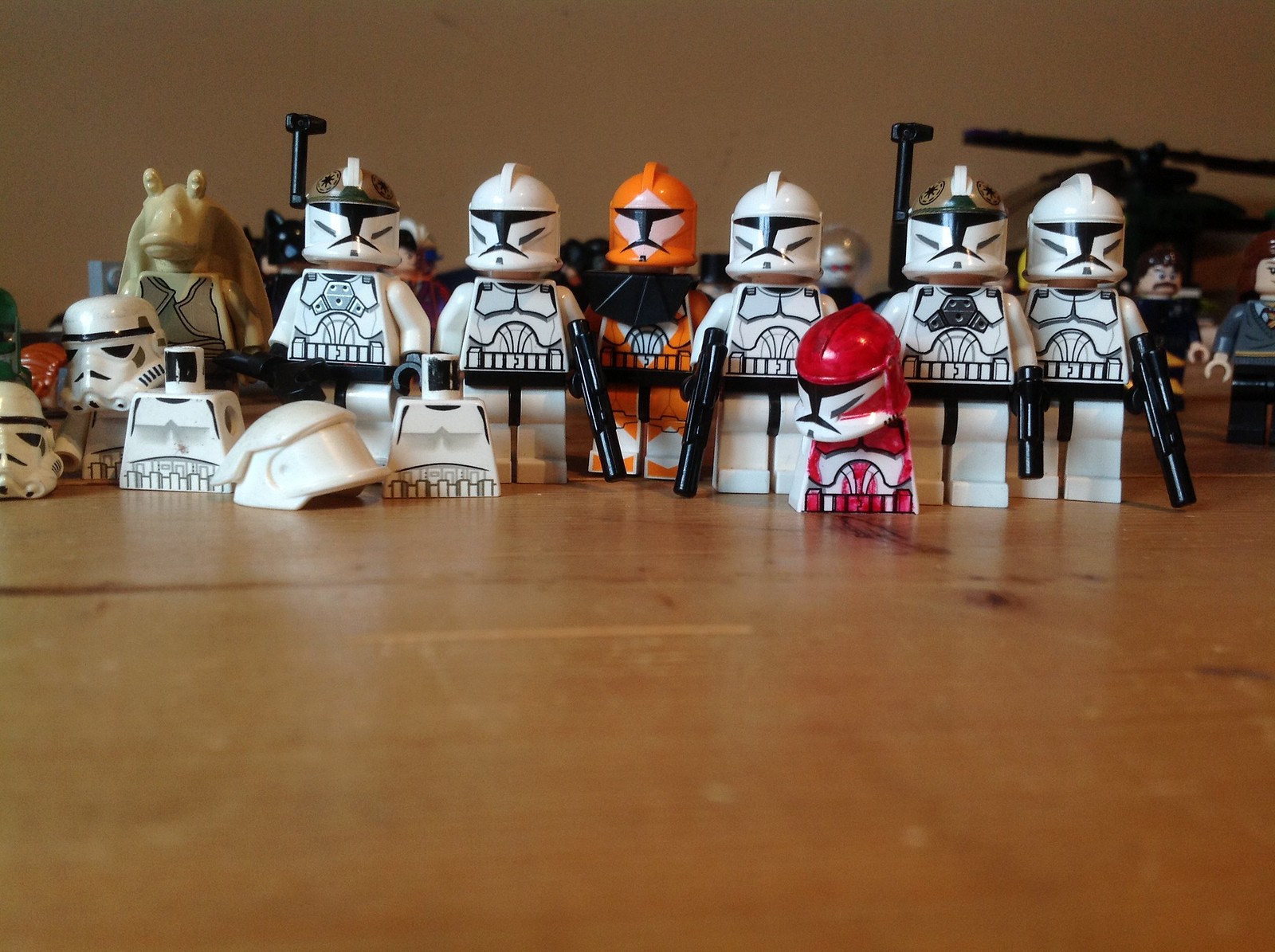The image captures a detailed ground-level view of various LEGO action figures arranged on a marked wooden table. The scene predominantly features multiple LEGO Star Wars figures, notably several Stormtroopers and Clone Troopers. The collection includes about seven to ten black-and-white Stormtroopers, some of which are disassembled with body parts scattered around. Among them is a distinctive orange, white, and black figure, as well as a shorter red, white, and black counterpart. Additionally, there's a light yellow frog-like figure that stands out among the characters. In the backgrounds are more LEGO figures resembling warrior-like humans, adding to the vibrant mix of colors, which primarily include brown, white, black, orange, and red. The back wall matches the tabletop in color, creating a cohesive backdrop devoid of any text or human presence.